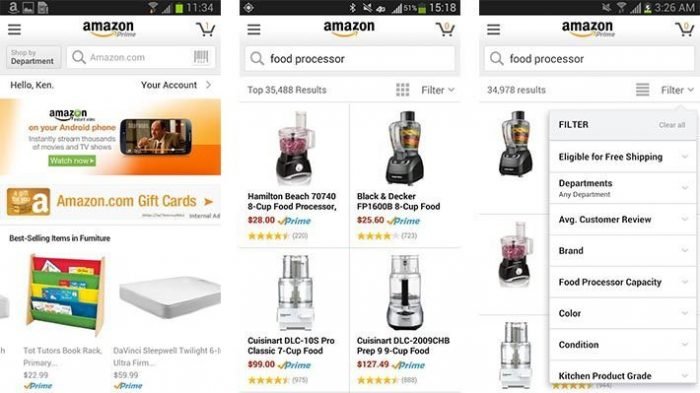This image features a three-panel collage of screenshots, each taken from the Amazon app on different cell phones. The screenshots are organized in three columns, placed side by side. 

- The leftmost screenshot displays Amazon's home screen, identifiable by the lack of a browser search bar at the top and the prominent "Amazon Prime" label. This screen highlights a personalized advertisement area suggesting various items and activities. Below the ad section, there is a segment labeled "Best Selling Items" featuring recommendations for furniture.
- The central screenshot, labeled "Amazon" without the "Prime," shows a search results page for "food processors." This page indicates there are over 35,000 results, though the visible portion of the screen displays only four different food processors.
- The rightmost screenshot, also labeled "Amazon Prime," depicts a similar search for "food processors." However, in this screen, the user has accessed a dropdown filter menu with various options for refining the search. This indicates an active engagement with sorting features to narrow down the extensive list of results.